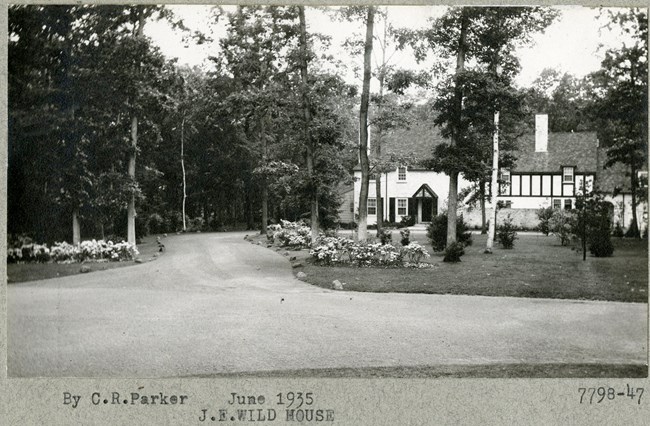This black-and-white photograph, taken outdoors during the daytime in June 1935 by C.R. Parker, captures an elegant Tudor-style home attributed to J.F. Wildhouse. The rectangular image, measuring approximately four to five inches wide and three inches high, is framed with a thin border and includes a light gray footer with typewritten labels: "By C.R. Parker," "June 1935," and "7798-47" on the far right. The stately two-story home is predominantly white with a possible stone foundation and features shutters on the windows, a slanted roof with chimneys on both sides, and a rectangular overhang above the entry door on the left. The well-manicured front yard showcases a lush grassy area, tall trees, and a flower-lined driveway that leads to the street. The organized layout and meticulous detail convey a sense of timeless elegance.